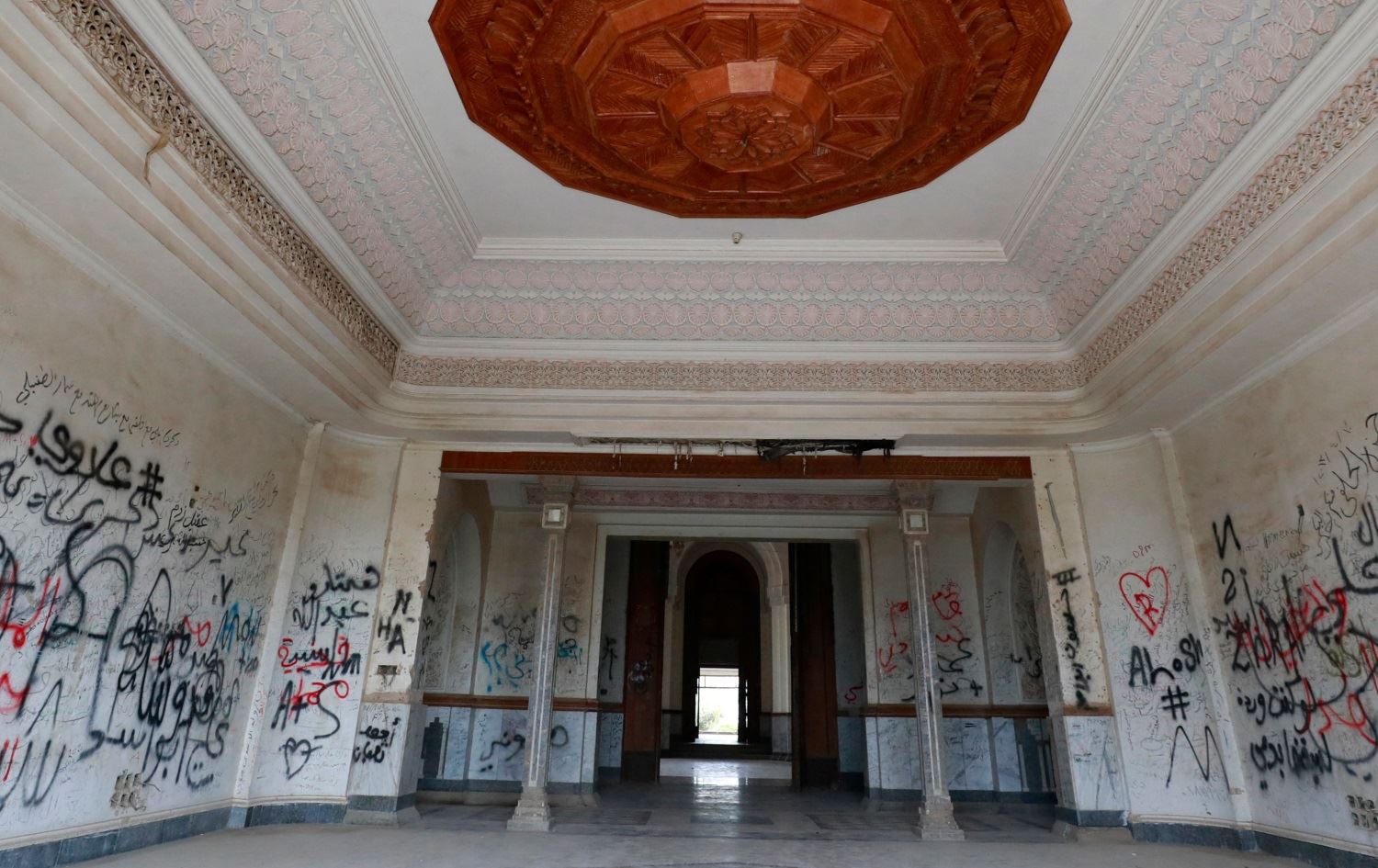The photograph captures the interior of a grand, cathedral-like room within a building. The space is large and empty, characterized by its untouched, intricately designed ceiling and the pervasive graffiti that covers the cream or light brown walls. The ceiling boasts an elaborate design with a prominent hexagonal-shaped, red centerpiece, surrounded by white, light pink, and brown decorative patterns. Two gray pillars stand on either side of the open front area, leading to additional rooms and spaces within the building. The walls, defaced with various forms of graffiti in predominantly black, red, and blue colors, contrast sharply with the room's otherwise lavish and expensive-looking features, including a beautiful copper chandelier. The overall atmosphere suggests a neglected elegance, marred by the inconsiderate scribbles of various artists.